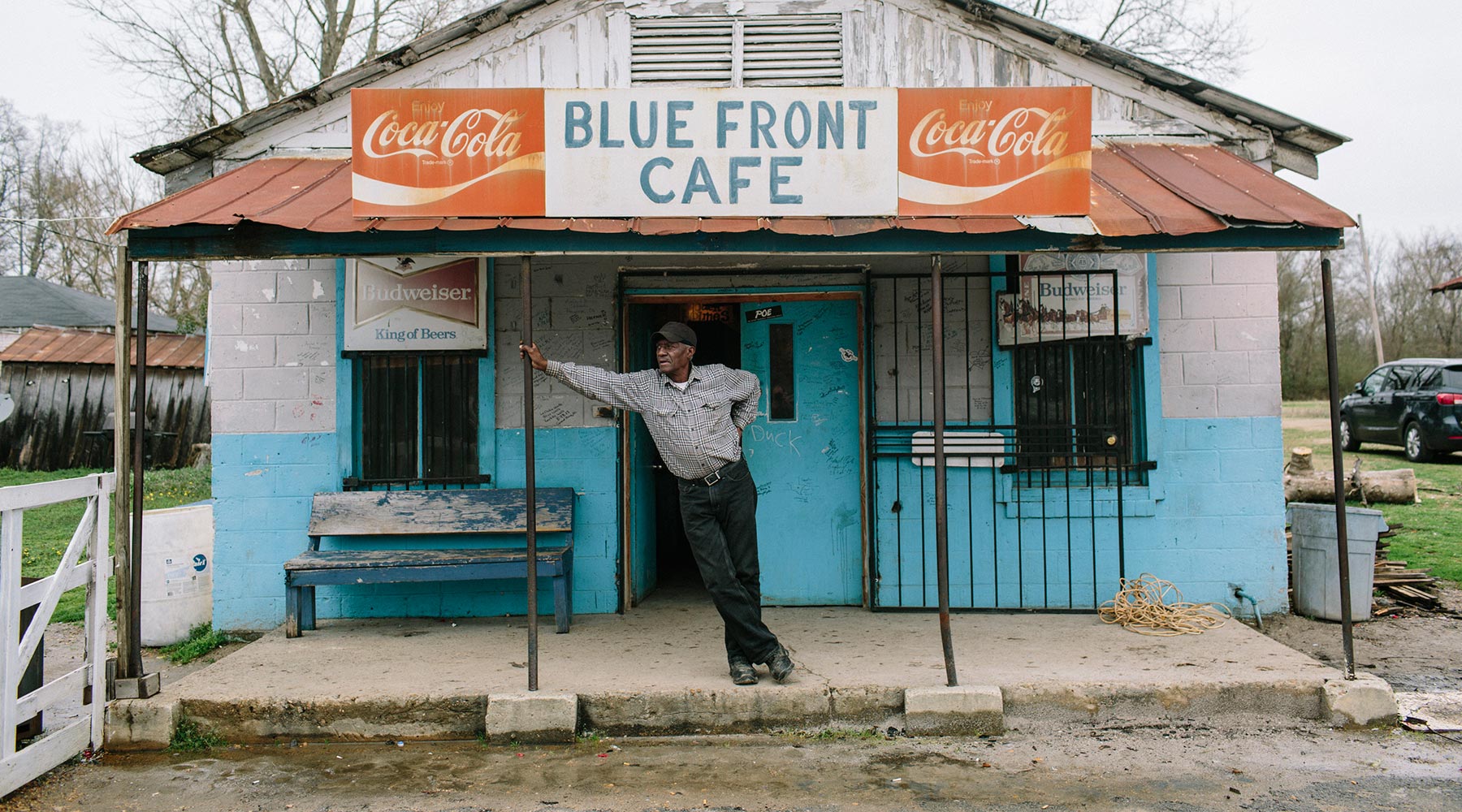In this photograph, a man is leaning on a black metal support pole in front of a run-down cafe. The building, which appears to be old and dilapidated, is constructed from large cinder blocks. The top half of the facade is painted light gray with some areas of chipping paint, while the bottom half and the double doors are painted an aqua blue. The double doors are set in a brown wooden frame, with the door on the left partially open. A large metal bar gate, normally covering the entrance, is currently swung open and resting against the front of the building. On either side of the doors are sizable windows framed in blue and protected by black metal bars, both adorned with similar Budweiser Beer advertisements.

Above the man is a weathered sign that reads "Blue Front Cafe" in blue letters on a white background, flanked by two worn Coca-Cola logo advertisements. The patio in front of the building is sheltered by a small overhanging roof made of corrugated rusty metal, supported by four black metal beams. A distinctive feature is a blue bench near the entrance, its paint mostly chipped away, revealing the raw gray wood beneath. The man, who is Black, stands with his legs crossed, leaning on the pole with his left arm fully extended, gripping it, adding to the scene's gritty, historic atmosphere.